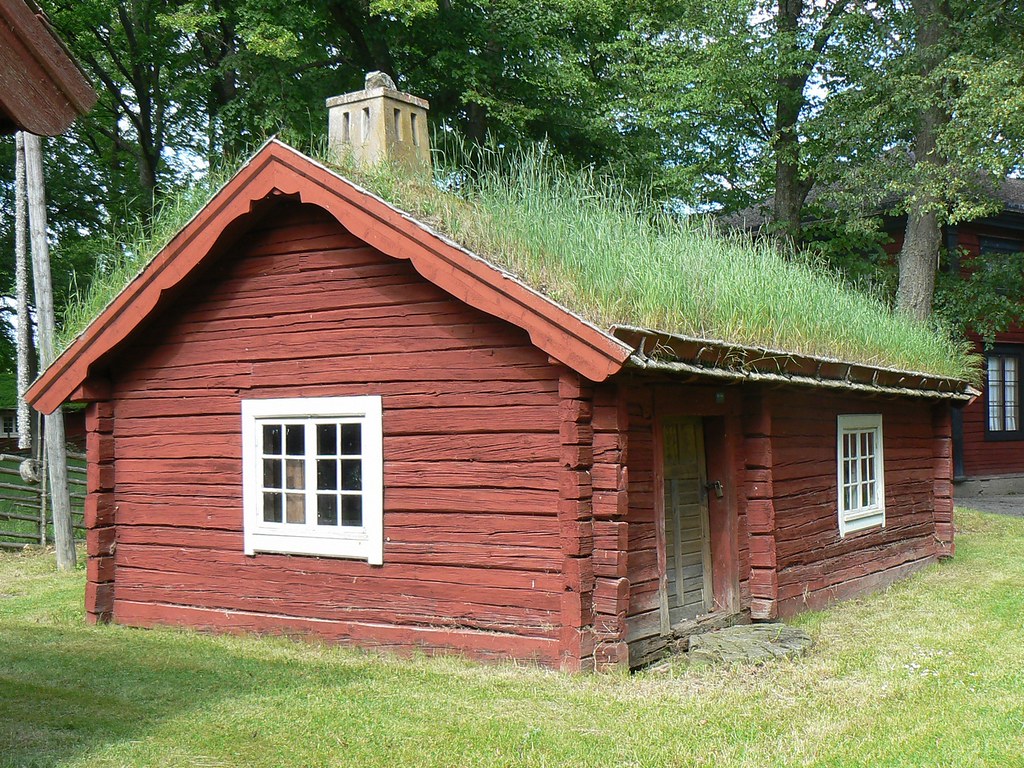This photograph depicts a small cabin with a rustic, thick wooden structure, prominently painted in reddish-brown hues. The cabin features two white-painted windows; one is clearly visible on the front facade while the other is on the side. The front door, also brown, is securely fastened with a padlock, and directly in front of the door, there is a noticeable rock resting on the green grass ground. Uniquely, the roof of the cabin has patches of green grass growing on it, and there is a light beige chimney sticking out at the top. To the right of the main cabin, partially visible, stands another building with red walls and a black-painted window. Tall trees with green foliage frame the scene and cast shadows over the ground, adding to the natural ambiance of the setting. Gray poles can be seen to the left, further enhancing the rustic charm of this picturesque landscape.